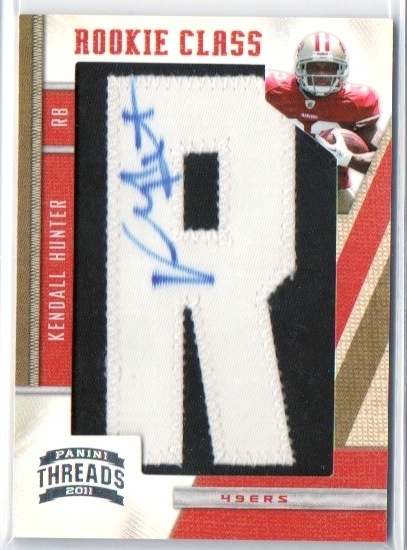This is a detailed photograph of a collectible football trading card, shown in portrait orientation and encased in a clear plastic protective sleeve with a thin transparent white border. The card prominently features several design elements and details. At the top left corner in bold red text, it says "Rookie Class," emphasizing the card's significance. To the right of this text, there is an action shot of Kendall Hunter, a football player, running with a football secured in his right arm. He is wearing a red jersey and a white helmet with two red stripes running down its center. The helmet has been variably described as gold, red, and white, indicating some reflective properties that might change colors under different lights. 

In the center of the card, a large white letter "R" is displayed on a black background. To the left of the "R," there is a blue signature, presumably belonging to Kendall Hunter. To the left side of the black box holding the "R," there is a vertical red rectangle containing white text that reads "Kendall Hunter, RB" in a bottom-up orientation. At the bottom portion of the card is a horizontal white banner with red text stating "49ers," representing Kendall Hunter's team, the San Francisco 49ers. Below and slightly to the left, there is another white rectangle indicating the card's series and year, which says "Panini Threads, 2011." Overall, the card’s colors—red, white, and a touch of gold—reflect the color scheme of the San Francisco 49ers.